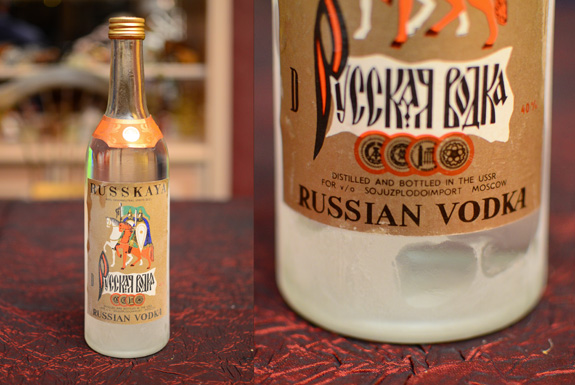This image depicts a vintage bottle of Russian vodka, presented in a split-frame format. The left side displays the full bottle, while the right side shows a close-up of its label and seals. The bottle features a clear, glass body transitioning to a cloudy white at the bottom, suggesting it might have been stored in a freezer. It is adorned with an orange ribbon around its neck and a brown label bearing the text "Russian Vodka" in black letters. The label also showcases an illustration of two knights on horseback, one orange and one white, framed by intricate detailing. Additional text on the right-side close-up reveals that the vodka was distilled and bottled in the USSR, with partial legible inscriptions that suggest it was for a specific brand in Moscow. The bottle is positioned on a table with a red tablecloth, against a blurred background that hints at a domestic or possibly bar setting.